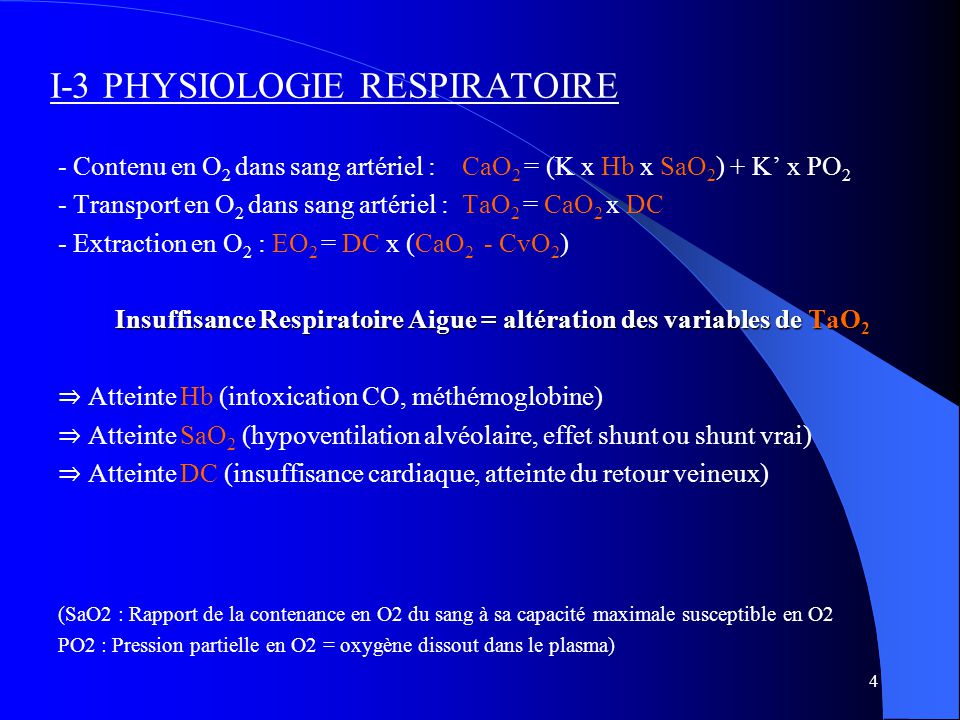The image is a detailed slide from a presentation, likely in French, focused on respiratory physiology. The background features a gradient blue, transitioning from a lighter blue on the left to a darker blue, almost black, on the right. The title at the top reads "I-3, Physiologie Respiratoire" in white text, suggesting a focus on respiratory physiology. The slide is filled with chemical and respiratory formulas, prominently CaO2 = K x Hb x SaO2 + K x PO2, indicative of oxygen content calculations. There are other formulas and definitions scattered throughout the slide, with some annotations in red, likely highlighting important points or symbols. A striking feature is a blue stripe on the right-hand side that tapers off into the background, adding a design element to the presentation. Overall, the slide combines a visually appealing gradient background with detailed and technical respiratory formulas, presented in French.